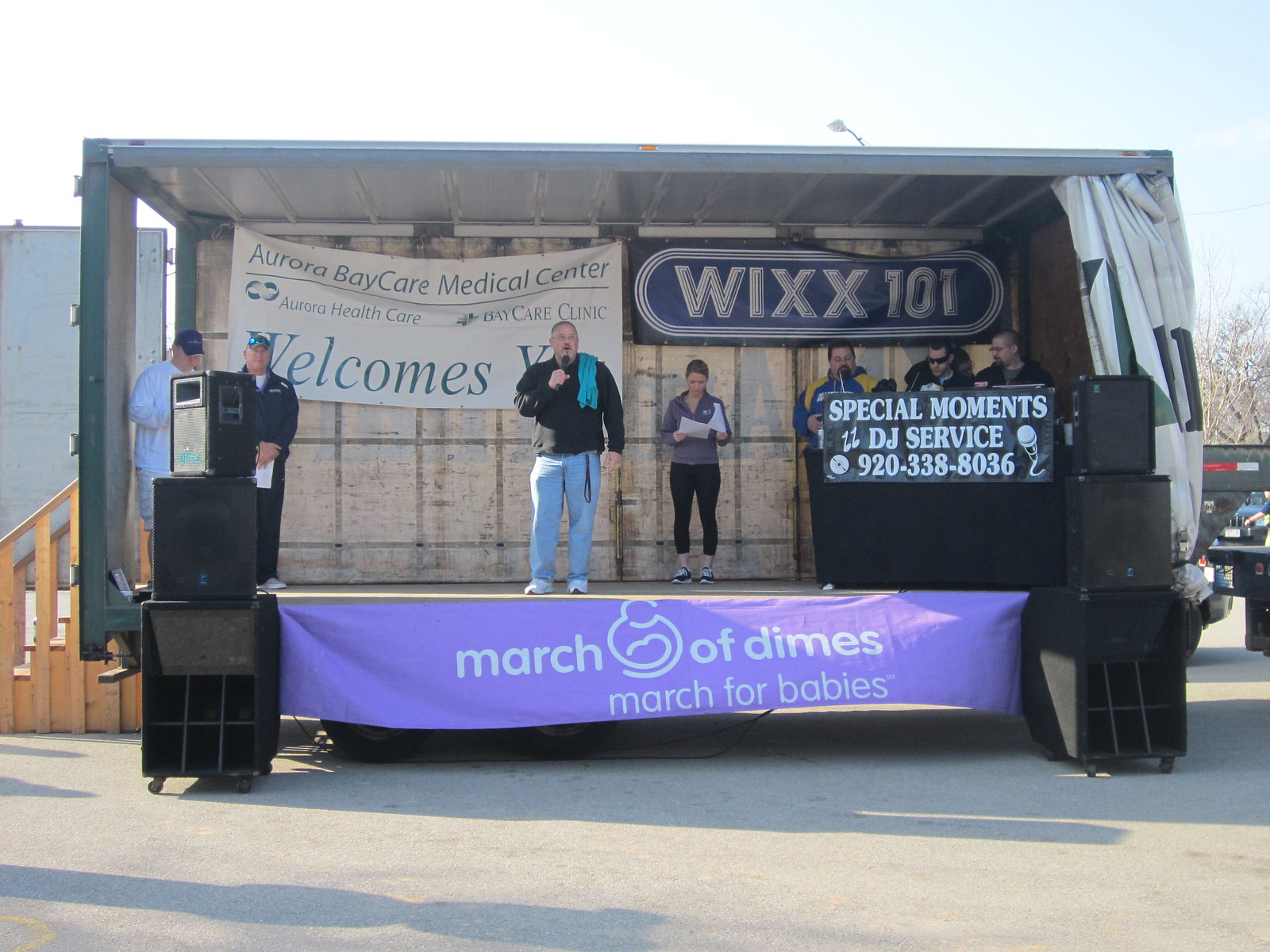This color photograph taken outside on a sunny day captures a mobile performance stage, turned from a trailer, with visible wheels at the bottom. The stage, which has walls around it and is open in the front, is decorated with various banners and signs. Prominently displayed at the bottom of the stage is a purple banner with white text and the outline of a mother with a baby, reading "March of Dimes March for Babies." The back wall features two banners: one from WICS 101, and another from Aurora BayCare Medical Center welcoming attendees.

On the stage, a central figure—a man in blue jeans and a black long-sleeve sweatshirt with either a blue shirt or towel draped over his left shoulder—stands holding a microphone. Behind him, a woman in athletic wear is looking at papers. To the left, two stacked speakers frame the scene, and several individuals add to the vibrant tableau. These individuals include one man in a white outfit with a baseball cap, and another man next to him in a blue long-sleeve shirt with black pants and sunglasses.

To the right of the stage, a booth or table with a sign reads "Special Moments DJ Service 920-338-8036," with three men positioned behind it, appearing to watch the action. Additional speakers are set up on either side of the platform, emphasizing the audio setup for the event. Completing the structure, movable wooden stairs are situated to the left, providing access to the stage.